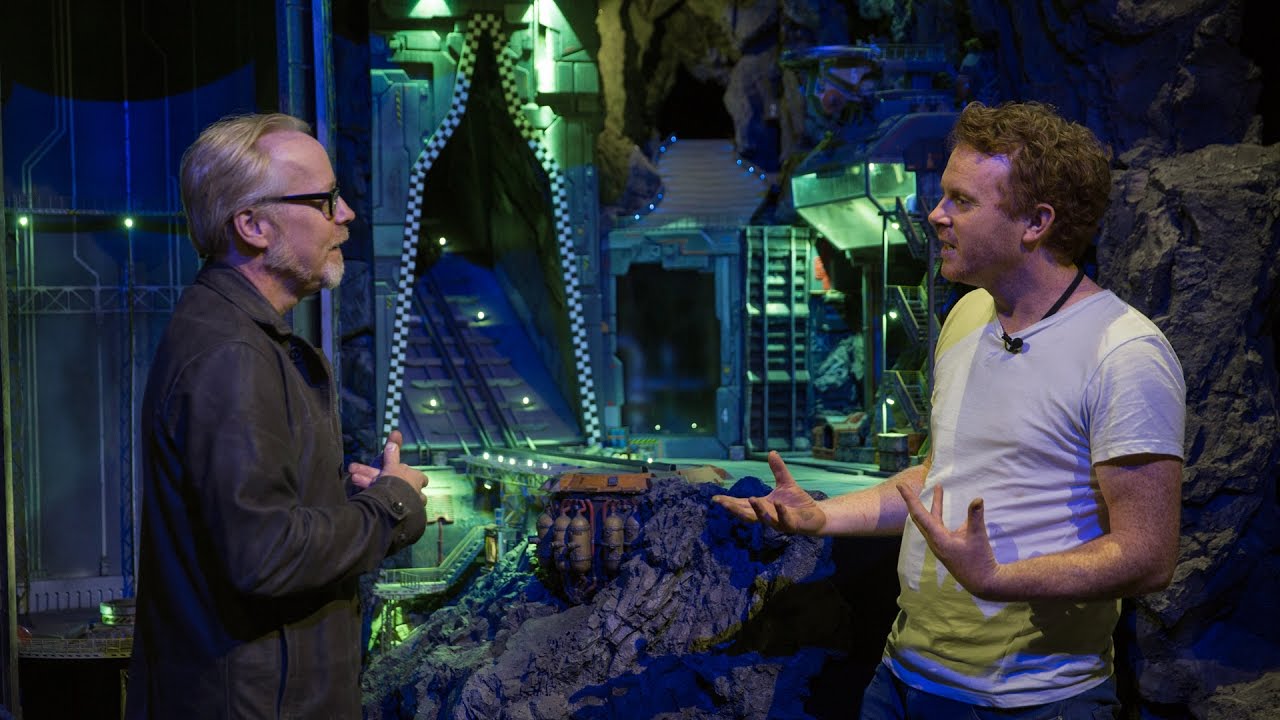In the photograph, set in what appears to be a visually striking, sci-fi themed studio, there are two men in conversation, possibly for a TV show or a movie scene. The man on the left side of the image is older with gray hair, wearing dark glasses and a dark leather-colored jacket, facing towards the younger man on the right. The younger man has short, curly blonde hair and is dressed in a white t-shirt, with his hands extended in front of him, palms up, as if explaining something; a microphone clipped to his shirt suggests he is speaking on camera. The background features a colorful array of lights in green, blue, and purple hues, and includes elements such as purple-colored rocks and a wooden door illuminated in purple light, contributing to the scene's otherworldly, futuristic atmosphere.